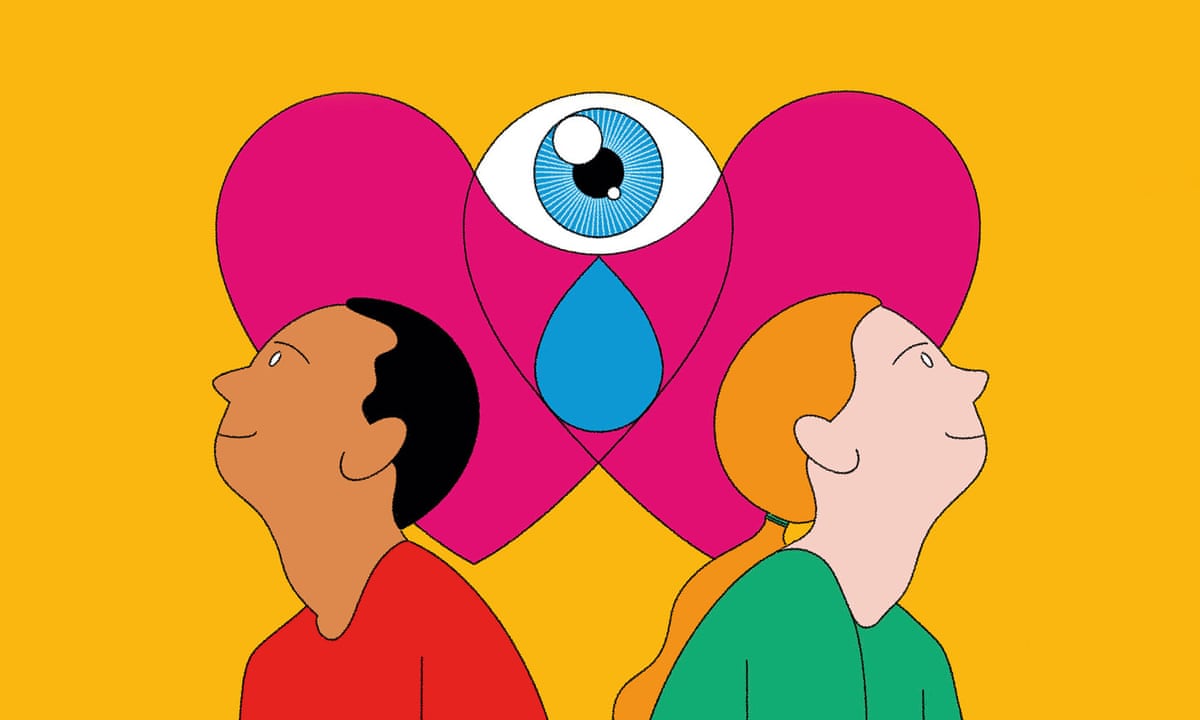This digital artwork features a detailed, cartoon depiction of a man and a woman presented from the shoulders up against a mustard yellow background. The man, positioned on the left, has a darker complexion, short black hair, and small white eyes, and is wearing a red t-shirt. He has a slight smile as he gazes upwards towards the top left of the image. Beside him, on the right, is a woman with fair skin, bright white eyes, and a subtle smirk on her face. Her long blonde hair is tied back into a ponytail that cascades down her back, and she is dressed in a light green shirt. Centered above them is an abstract, elongated heart shape that houses a prominent, large blue eye with a black pupil and white sclera. This heart-eye formation is pink and features wings on either side, and directly beneath the eye is a single blue teardrop. The composition richly includes multiple colors: red, green, pink, blue, white, and the distinctive mustard yellow background. The two figures are not interacting with each other but seem to be looking away, perhaps contemplating or dreaming, adding an element of introspection to the scene.